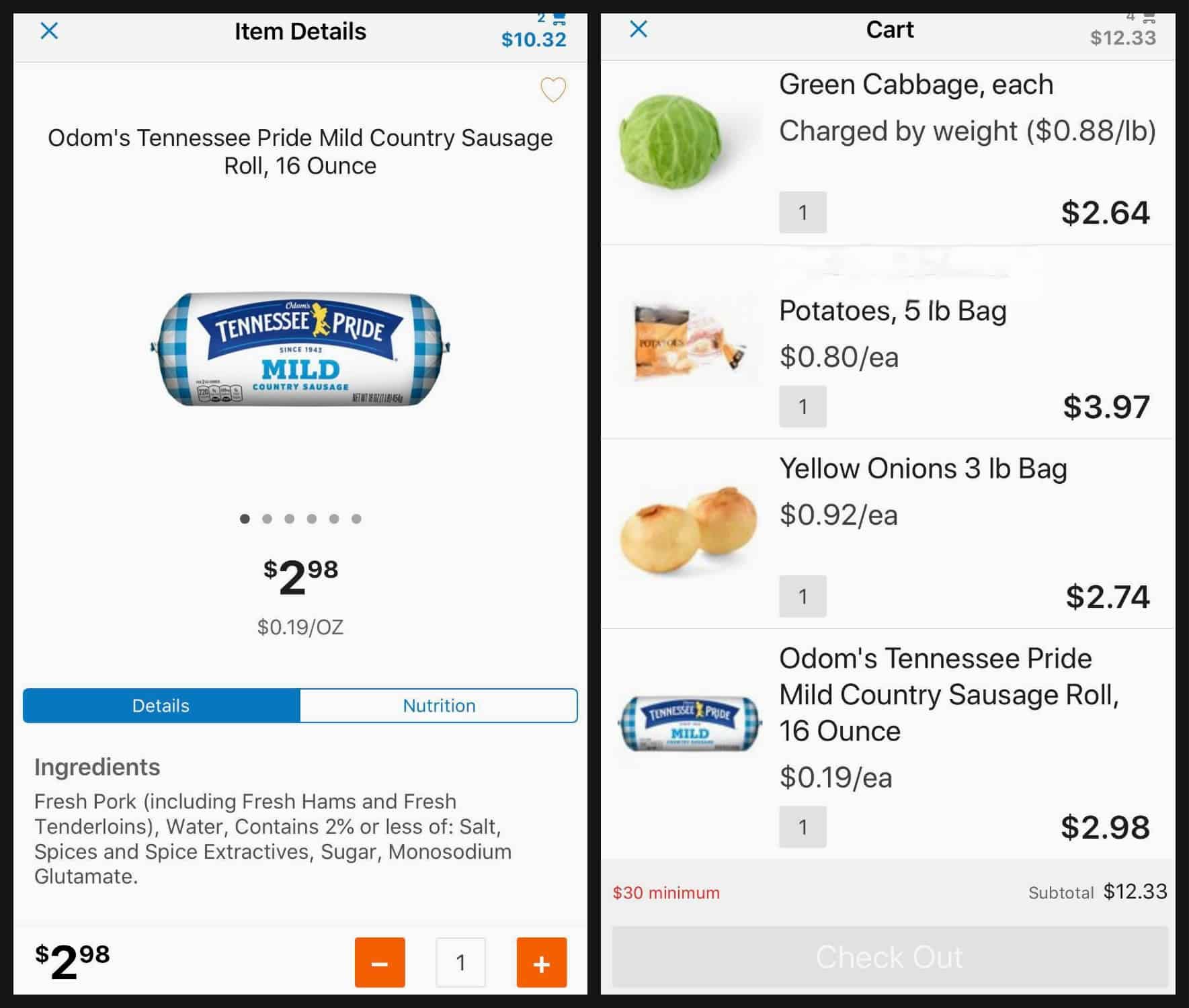In this composite image, we see two screenshots presented side by side. The left screenshot displays promotional information for "Odum's Tennessee Pride Mild Country Sausage Roll, 16 ounces," priced at $2.98, which translates to 19 cents per ounce. Detailed ingredient information is provided, listing fresh pork (including fresh hams and fresh tenderloins), water, and 2% or less of salt, spices and spice extractives, sugar, and monosodium glutamate.

The right screenshot features a grocery bag with a detailed itemization and prices: green cabbage for $2.64, a 5-pound bag of potatoes for $3.97, a 3-pound bag of yellow onions for $2.74, and the aforementioned sausage.